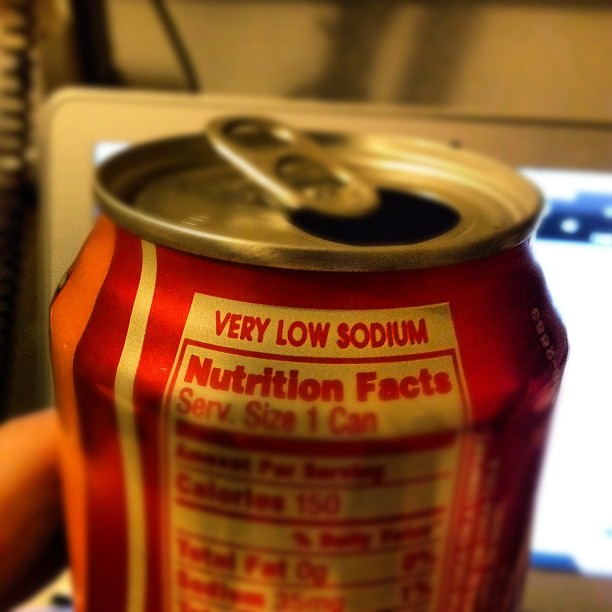This photograph captures a close-up of an open, shiny red aluminum soda can with a pull-tab top. The can features a vertical white stripe down the side and a hint of orange coloring on the left. Prominently displayed on the silver top of the can is a white rectangle containing nutritional information printed in red text. Although some lines are blurred, it states "Very Low Sodium," "Nutrition Facts," "Serving Size: 1 Can," "Calories: 150," and "Total Fat: 0g," among other details. In the background, an illuminated computer monitor or possibly an iPad can be seen, along with a white wall. The image also shows at least one finger holding the can, underscoring the beverage as the focal point amidst a slightly blurred but distinguishable digital workspace.